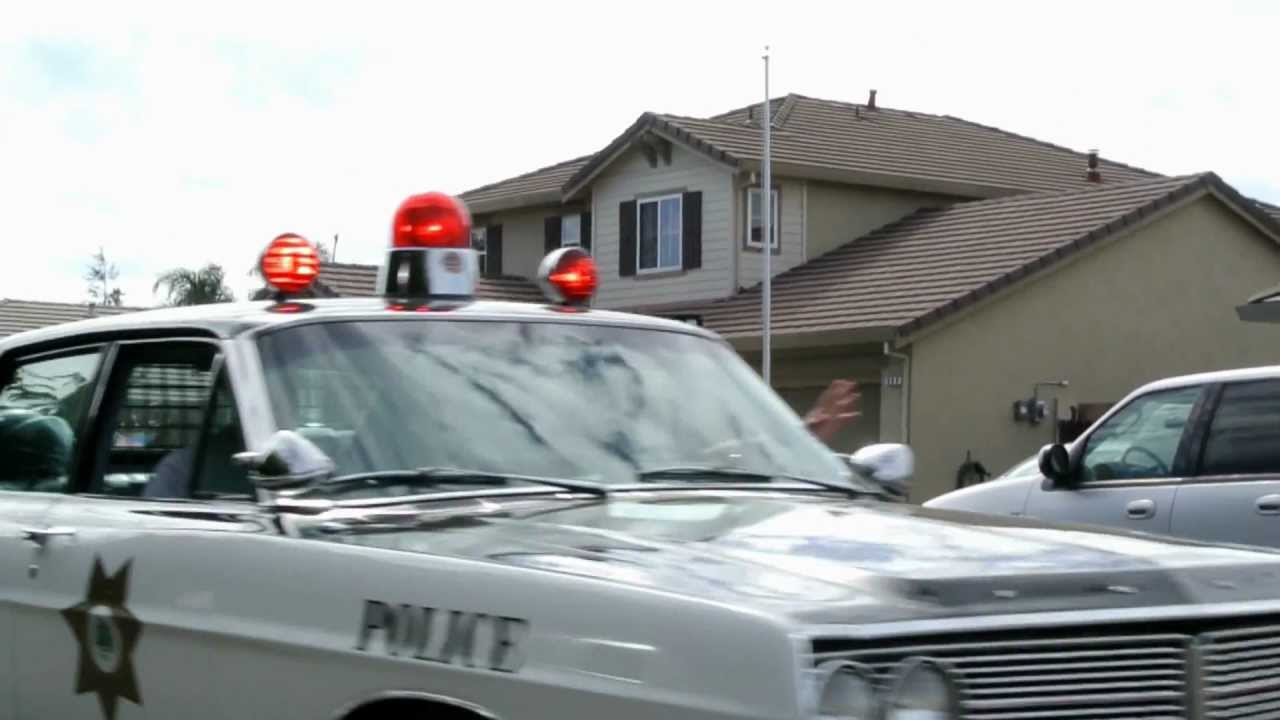The photograph captures a dynamic scene featuring an old-fashioned, gray police car traveling down a neighborhood road. The car, with the word "POLICE" emblazoned on its side and a star-shaped emblem on the door, has three red lights atop its roof and presents a slightly blurred image, suggesting movement. Through the driver's side window, a policeman's hand extends outward, possibly waving, while another individual is faintly visible in the passenger seat. Flanking the police car on the left is a parked silver sedan, facing the opposite direction. The scene is set against a backdrop of a two-story, beige house with a gabled roof, which also features a flagpole without a flag. The sky appears somewhat sunny and cloudy, highlighting the daytime setting of this residential area.